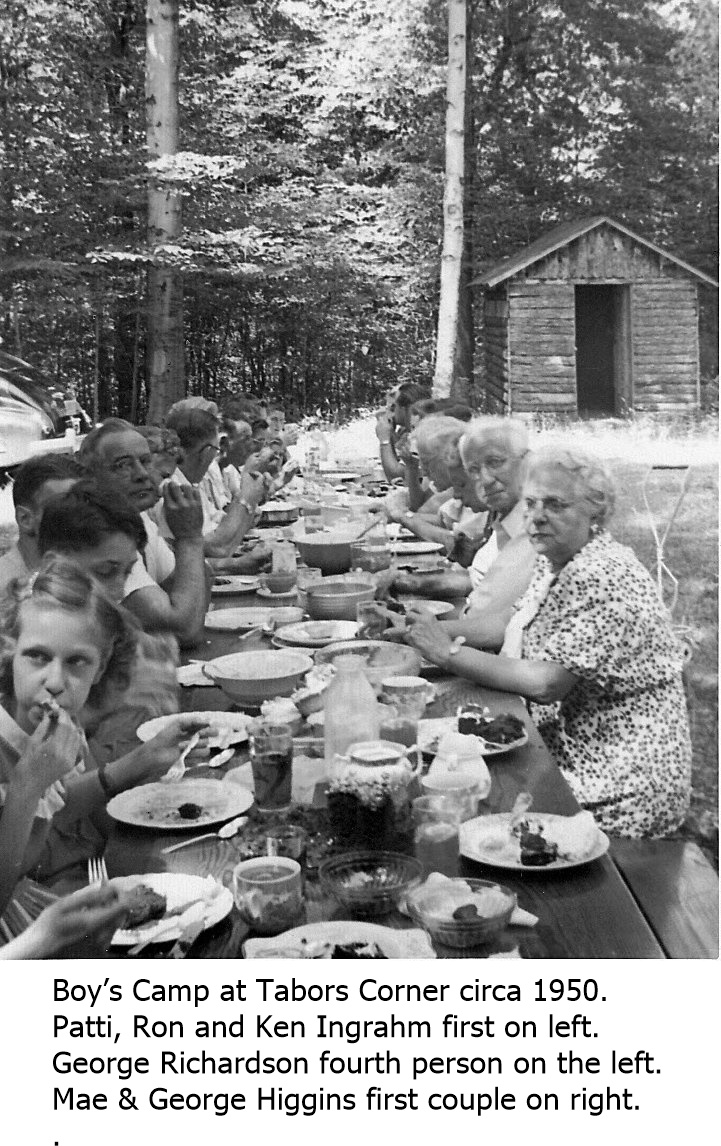The black-and-white photograph, likely taken circa 1950, captures an outdoor setting at the Boys Camp at Tauber Center. At the center of the image is a large rectangular table, adorned with several bowls, cups, spoons, and silverware, indicating a communal dining setup. The table is surrounded by people of various ages, with elderly individuals predominantly on the right side and younger people on the left. The background features dense trees and a brick building on the upper right, signifying a serene and wooded camp environment. The caption at the bottom of the image identifies several individuals: Patty, Ron, and Ken Ingram as the first on the left, George Richardson as the fourth person on the left, and May and George Higgins as the first couple on the right. The scene, rich in historical context, is a vivid glimpse into mid-20th-century camp life.